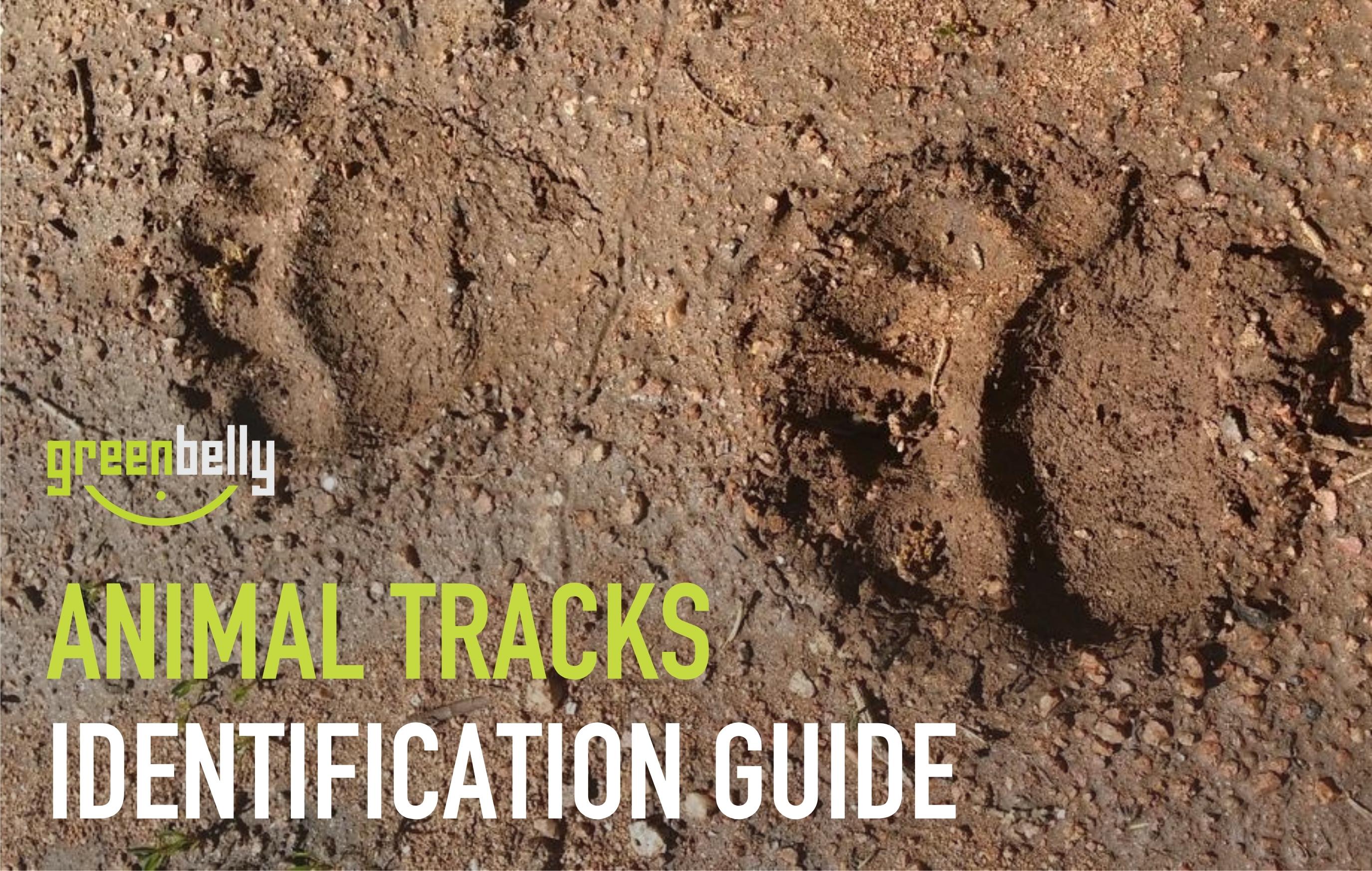The image depicts a pair of animal footprints set in a background of brown dirt or soil. The left print is slightly smaller than the right, and both are oriented with the toes pointing left and the heels to the right. In the bottom left corner of the image, the phrase "green belly" is displayed in lowercase letters, with "green" in a yellowish-green color and "belly" in white. Below this text is a semi-circular line and a dot. The phrase "ANIMAL TRACKS" appears larger in an all-cap sans-serif yellowish-green font, with "IDENTIFICATION GUIDE" written beneath it in all-cap white font. The entire text layout seems to resemble a cover or a section from a guide or resource dedicated to identifying animal tracks, possibly bear tracks, as inferred from the footprints. Some falling leaves can also be noticed below the letters 'E' and 'N' in the word 'IDENTIFICATION'.